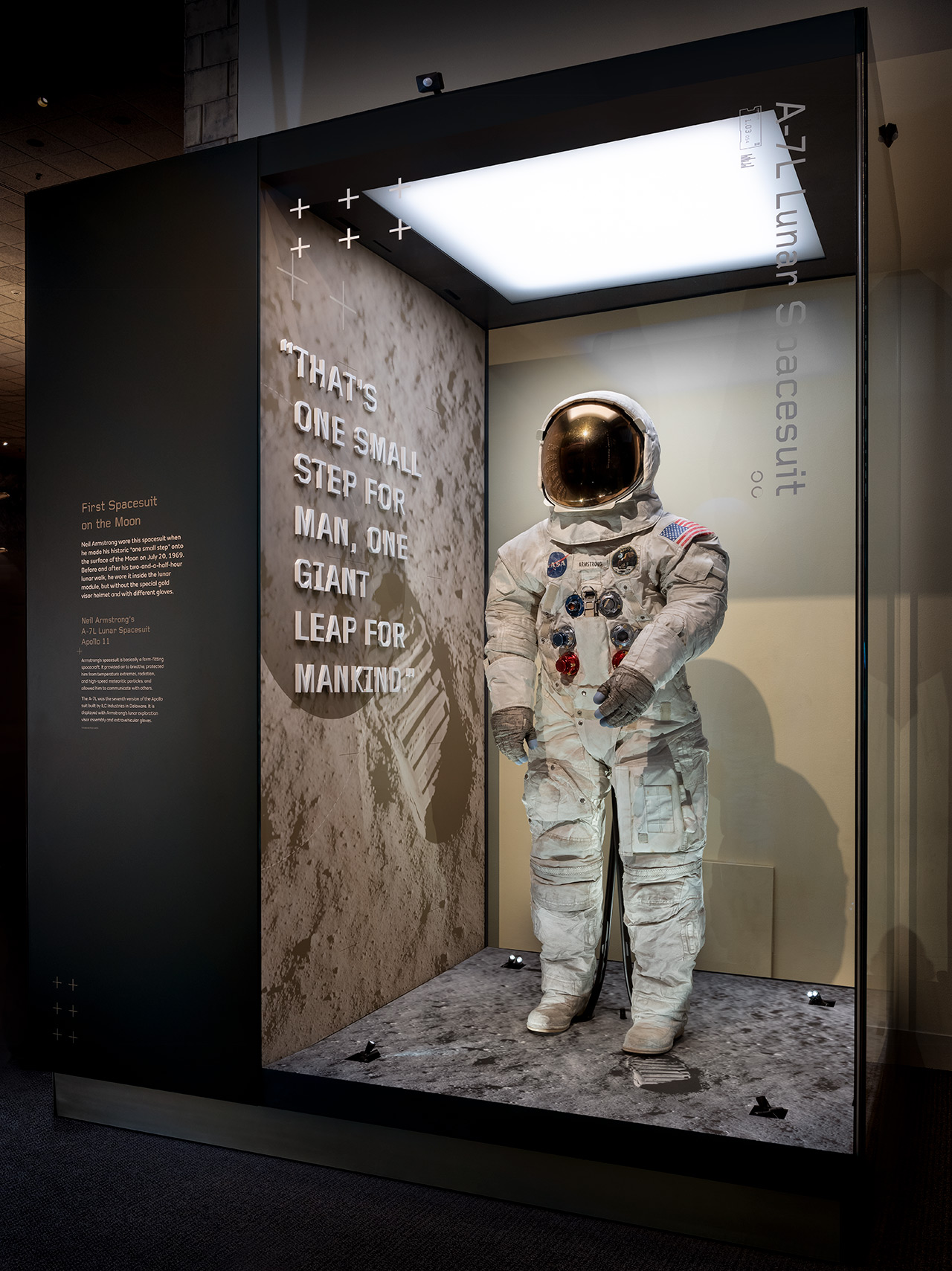The image depicts a detailed museum exhibit showcasing the first spacesuit worn on the moon. The spacesuit, identified as the A-7L Lunar Spacesuit worn by Neil Armstrong, is encased in a glass enclosure with a black border. The floor of the enclosure is designed to resemble the moon's surface, complete with grey craters, and a large white light shines down on the exhibit, enhancing its display.

Inside the enclosure, the spacesuit stands prominently with its distinctive features: a black visor, a white suit adorned with a NASA logo (a blue circle with the word 'NASA' and a red line through it), an American flag on the shoulder, several valves, and grey gloves. Near the top right corner of the glass booth, the words "A-7L Lunar Spacesuit" are etched vertically, while the left side contains a black information panel that includes a description and context about the spacesuit and the moon landing.

Additionally, the left wall of the enclosure features a photograph of the lunar rover on the moon and 3D letters displaying the iconic quote, "That's one small step for man, one giant leap for mankind," in white. The exhibit is meticulously crafted to provide an immersive and educational experience, commemorating mankind's monumental achievement in space exploration.